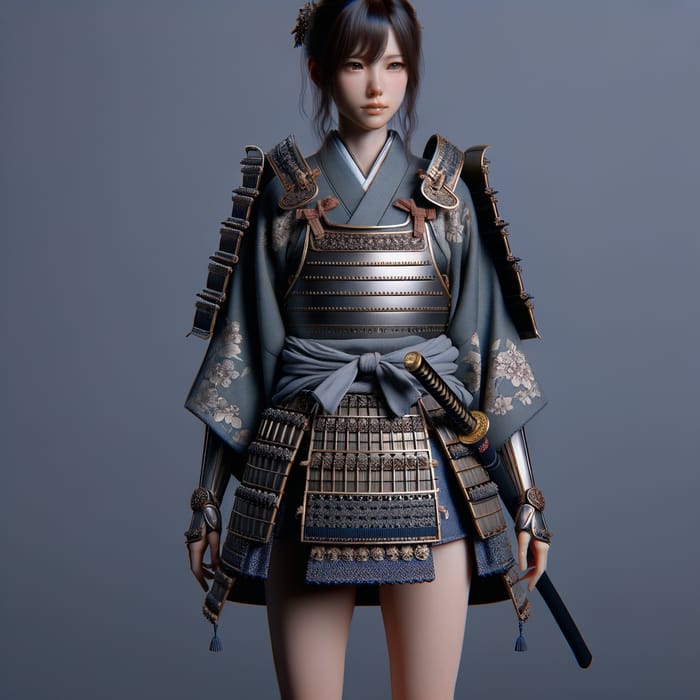In a seemingly computer-generated or AI-produced image, likely intended for a video game, an Asian female character stands against a dark gray background. She appears young with shoulder-length black hair, with some of it neatly tied in a bun at the back. Her bangs slightly cover one of her calm, expressionless eyes as she gazes off to the side. She is dressed in detailed samurai armor featuring bronze and black plated chest armor, shoulder straps, and an armored skirt with metal plating on the sides and front. A gray kimono with a tan flower motif on the sleeves lies underneath the armor. It stops short above her knees, revealing her bare legs. She also sports fingerless metal gloves on her arms. A gray sash belts her waist, holding a samurai sword with a black handle and a bronzed end, sheathed in a scabbard hanging on her left side. Tassels hang along the bottom of her armored skirt, contributing to the intricate and realistic appearance of her warrior attire despite the image's digital or possibly cosplay nature.